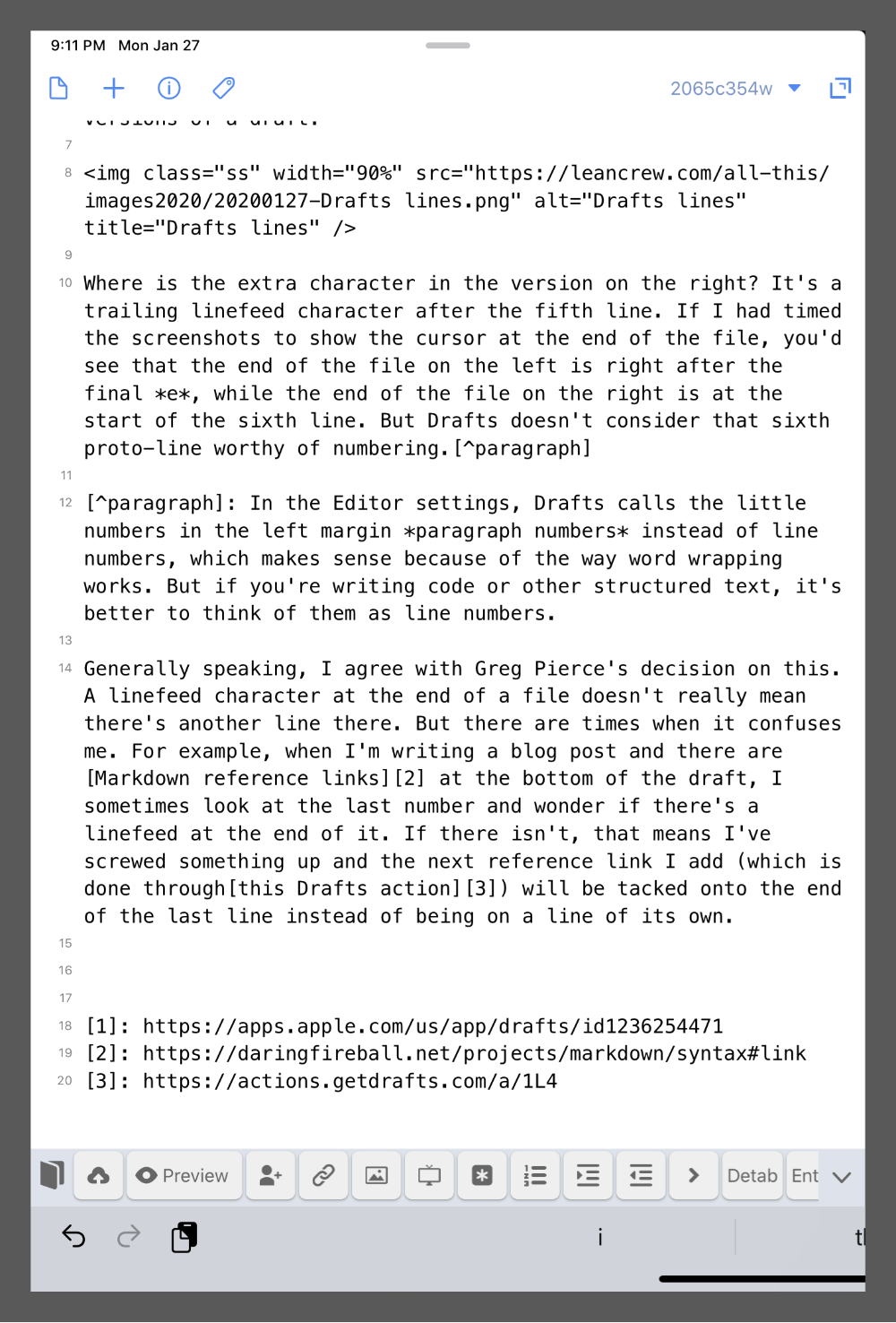A screenshot of a generic document reader app on an iPhone, displaying a plain-text document with basic word processing features. The text is organized into multiple paragraphs, although each paragraph appears to be treated as a single, long line by the software, with automatic text wrapping for easier reading. Along the left margin, there are numbers incrementing sequentially, which may denote line numbers or a similar reference system. The text includes a note expressing agreement with a decision made by Greg Pierce. The interface of the app is simple and uncluttered, focusing primarily on the readability of the document.